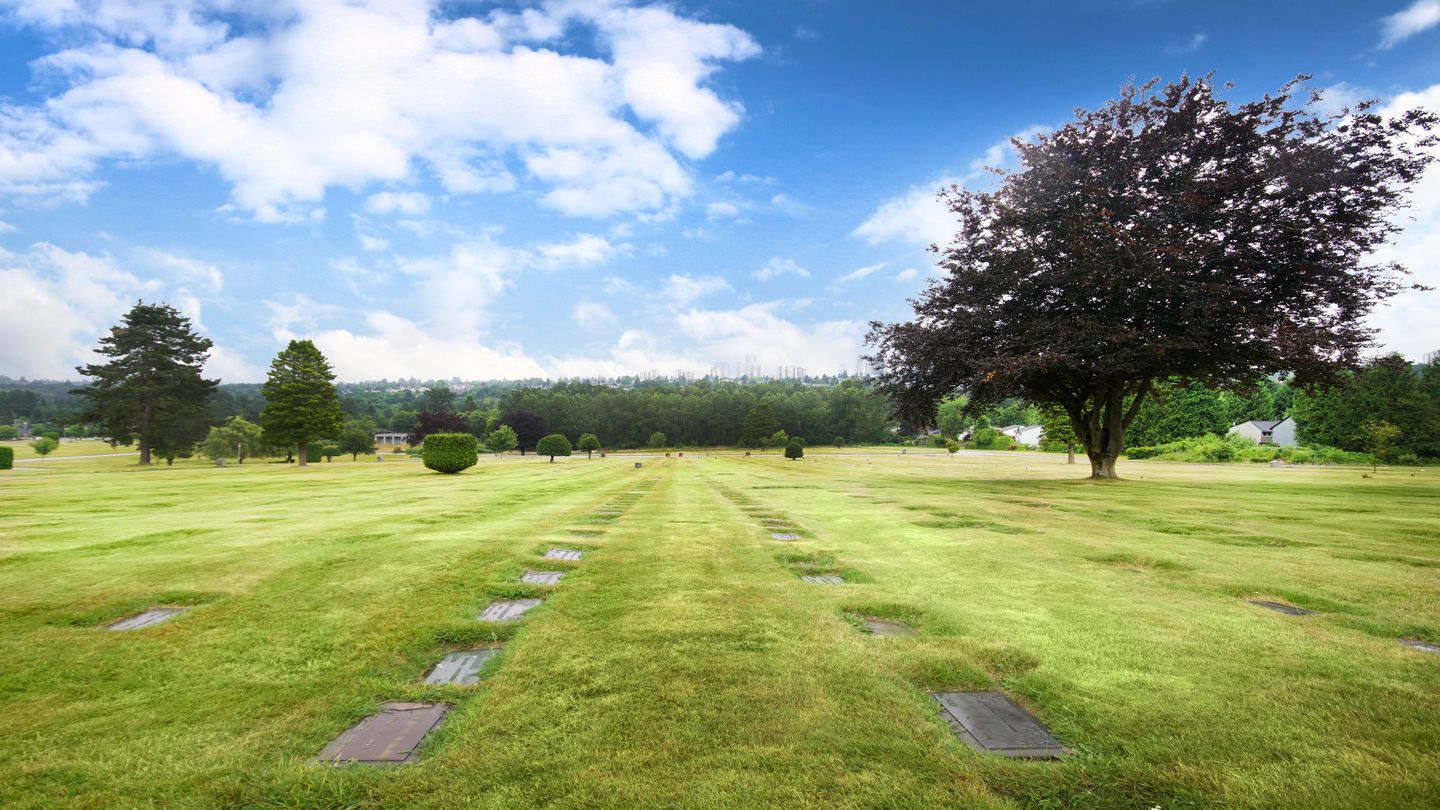The photograph presents a serene, expansive graveyard during the daytime. The cemetery stretches far into the distance, featuring neatly arranged rows of rectangular grave markers that lie flat on the ground, spaced evenly by green grass. The graveyard is adorned with several large trees, including two pine trees positioned on the left, and a notably closer tree on the right exhibiting shades of pink and green. Additional greenery in the form of trimmed bushes and shrubs punctuates the landscape. The thick grass carpeting the cemetery is a light green color. In the far distance, a dense line of green trees marks the horizon, with a forest beyond. Above, the sky is a clear blue with substantial white cloud coverage, adding to the tranquil atmosphere. In the background, one or two houses can be spotted, although the graveyard itself is devoid of people.